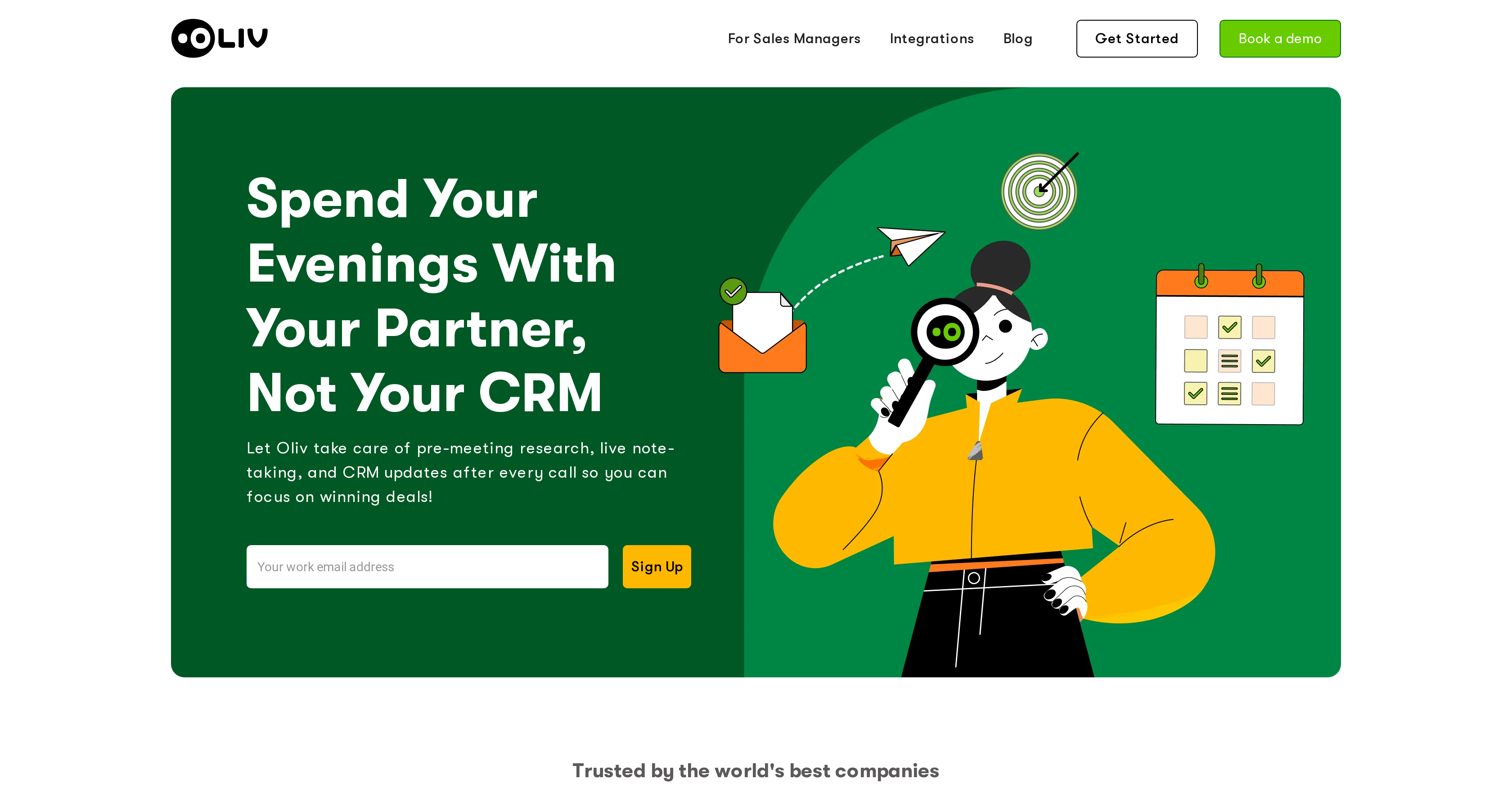The top section of the image features a black oval, within which sits a small white circle on the left and a larger white circle on the right. The larger circle has a black dot in its center. To the right of this oval, the text "LIV" is displayed in bold, black capital letters. Adjacent to it, on the right, there is text that reads "For Sales Manager Integration Blog." Below this text are two buttons: a white rectangle with the words "Get Started" and a green rectangle labeled "Book a Demo."

The lower part of the image has a dual-colored background: dark green on the left and light green on the right. It features an illustration of a woman wearing a long-sleeved orange shirt and black jeans. She is holding a magnifying glass up to her face. Accompanying the illustration are various icons: an envelope with a green checkmark, a paper airplane, a target with a bullseye, and a calendar.

On the left side of the lower section, there is text that reads, "Spend your evening with your partner, not your CRM. Let LIV take care of pre-meeting research, lab note-taking, and CRM updates."